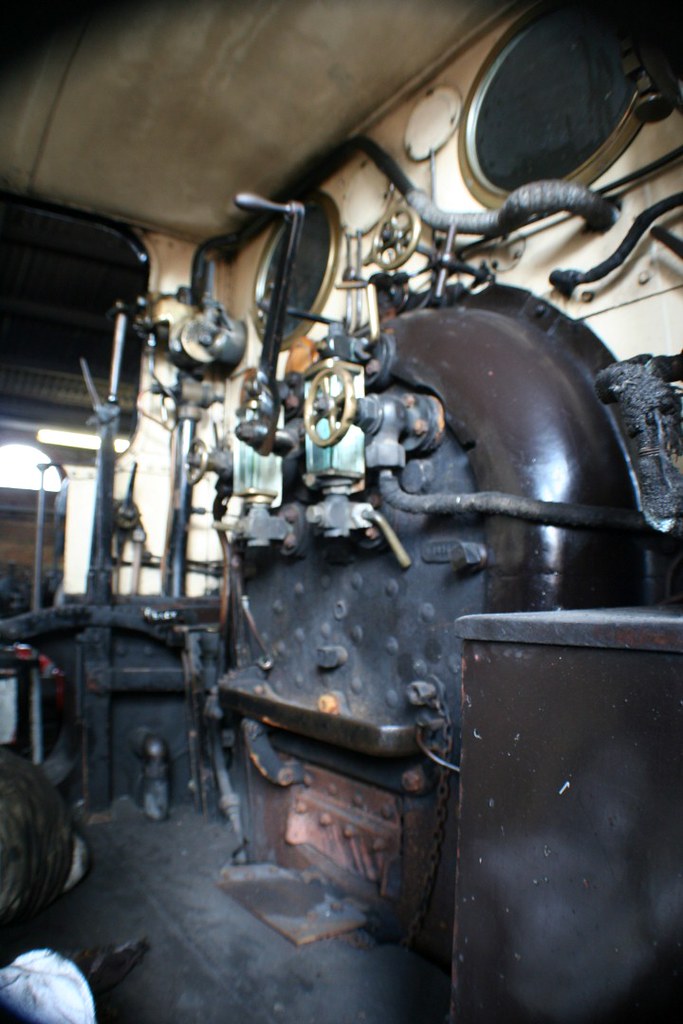The photograph, taken in portrait orientation, captures an aged and weathered interior of an engine room, possibly on a ship. The focus is on a central, dark-colored metal machinery system. At the bottom, the machinery features a lighter brown, openable grill or furnace door, likely used for feeding coal or wood into the boiler for heating. Above this, a complex arrangement of control valves, knobs, and levers is visible, with various pipes extending upward and connected to the surrounding structure.

The walls behind this intricate machinery are cream-colored, adorned with two brass-bezeled porthole windows to the right. These round windows suggest a maritime environment. To the upper left of the machinery, there is a rectangular window set high on the wall. The overall scene is dimly lit, enhancing the sense of age and historical realism, characteristic of photographic representationalism.